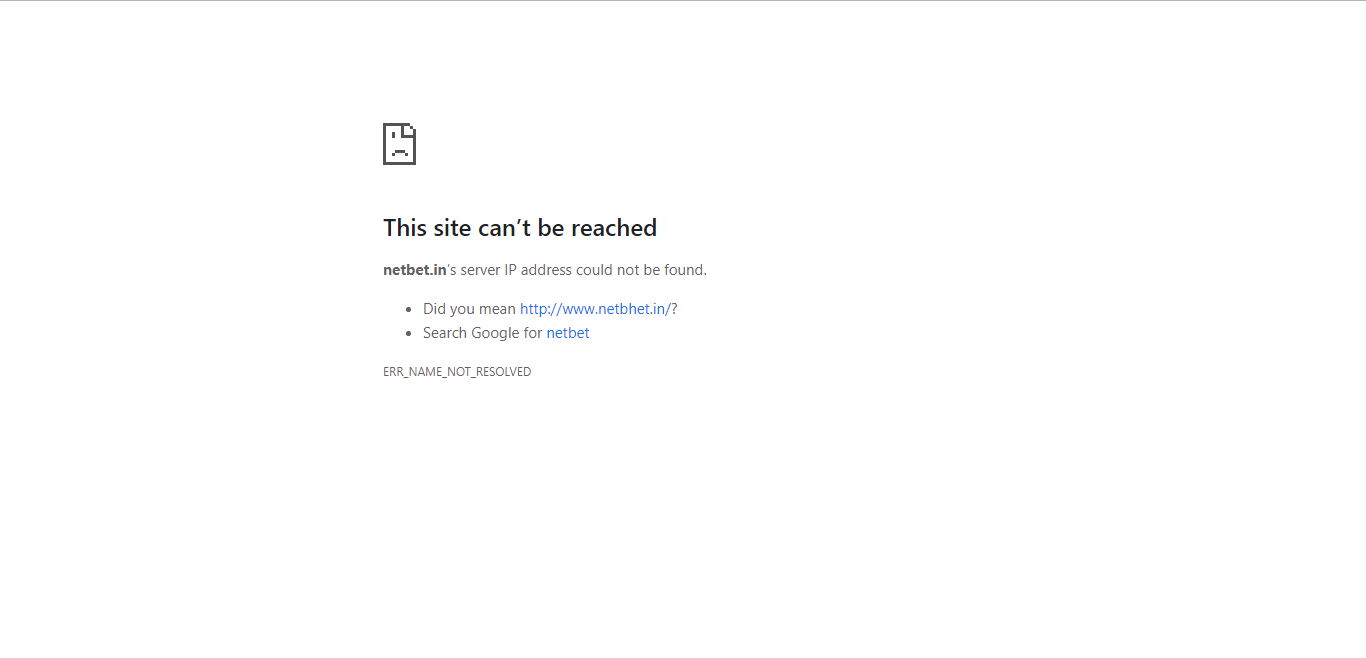**Caption:** 

This image is a screenshot of a webpage displaying an error message, likely captured on either a desktop or mobile device. The page has a clean and minimalist aesthetic, with a pure white background and ample negative space, disrupted only by a thin, dark grey line running horizontally across the top of the page.

The central element of the screenshot is the error message itself, positioned slightly above the center of the page both horizontally and vertically. At the top left corner of the error message is a small icon of a folded page with a corner turned down on the top right, featuring an anthropomorphized sad face with a single eye on the left and a frown at the bottom.

Directly beneath the icon, in large black sans-serif text, the message reads: "This site can't be reached." The next line, in slightly smaller text, states, "netbet.in's server IP address could not be found." The domain 'netbet.in' is bolded for emphasis while the rest of the text is standard.

Following this, there are two bullet points providing further suggestions. The first bullet point asks, "Did you mean http://www.netbhet.in?" The second bullet point suggests, "Search Google for netbet," with the word 'netbet' displayed in blue, indicating a clickable link.

Concluding the message, at the very bottom, in plain text, is the technical error code: "ERR_NAME_NOT_RESOLVED."